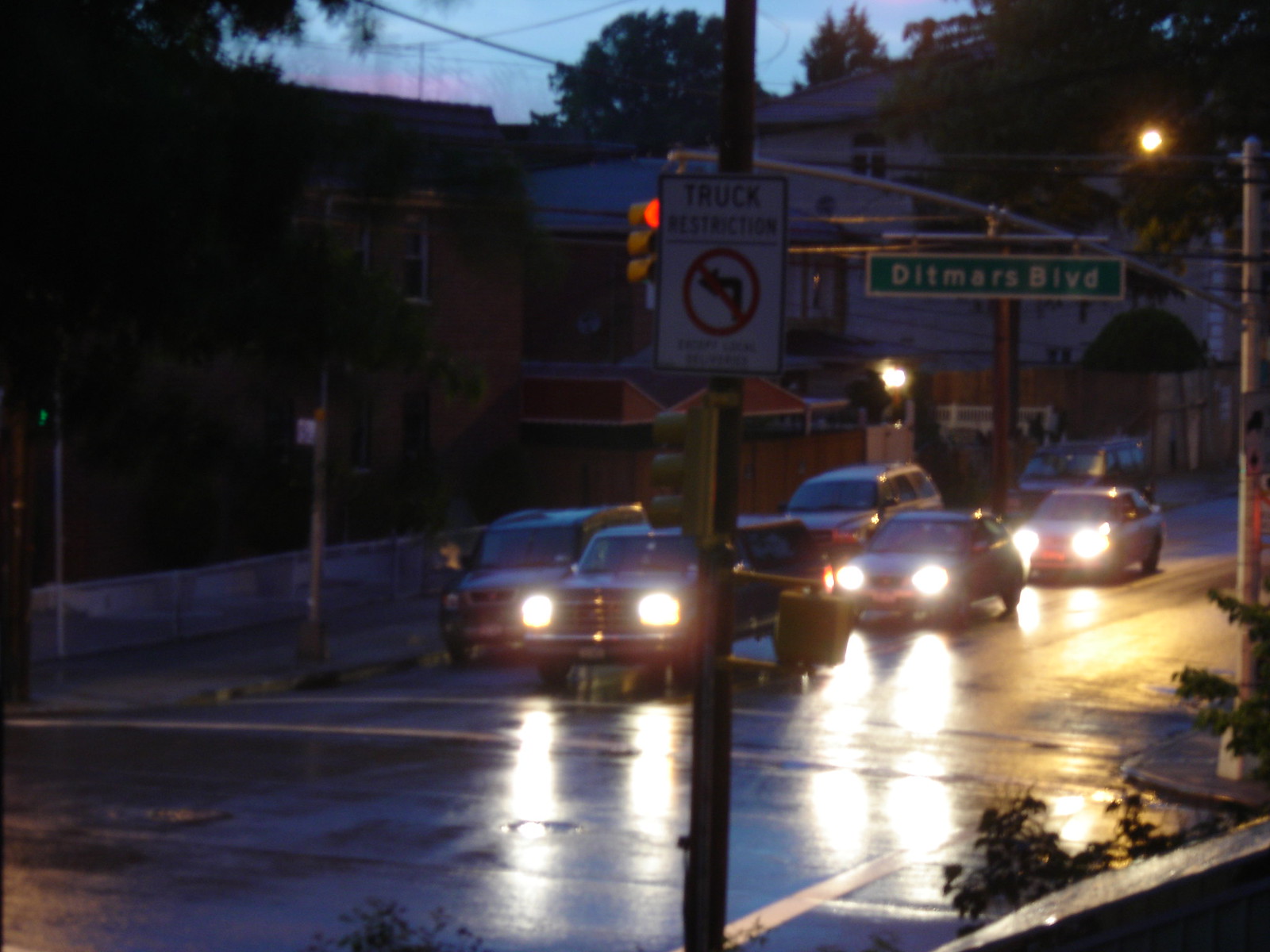This detailed image captures a night or early dusk scene on Dittmar's Boulevard, featuring a series of five cars on a wet, shiny road, possibly hinting at recent rainfall. Three cars, their headlights casting beams of light onto the gray asphalt, are lined up at a red light in the center of the frame, while three more cars appear to be parked adjacent to a sidewalk running through the middle of the picture. 

In the foreground, a vertical pole prominently displays a "Truck Restriction" sign, marked by a red ring, a black arrow pointing left with a red line through it, indicating no left turn for trucks. To the right of this pole, dark green leaves suggest nearby bushes. On the left-hand side, a range of buildings—some brick, some a lighter color—are visible, framed by an array of trees and dark foliage. Above these, a patch of deep blue sky peeks through, adding to the dim yet tangible light. The scene is set in a residential neighborhood, denoted by the presence of smaller buildings and fences, and illuminated faintly by streetlights and the dying light of dusk or early evening.